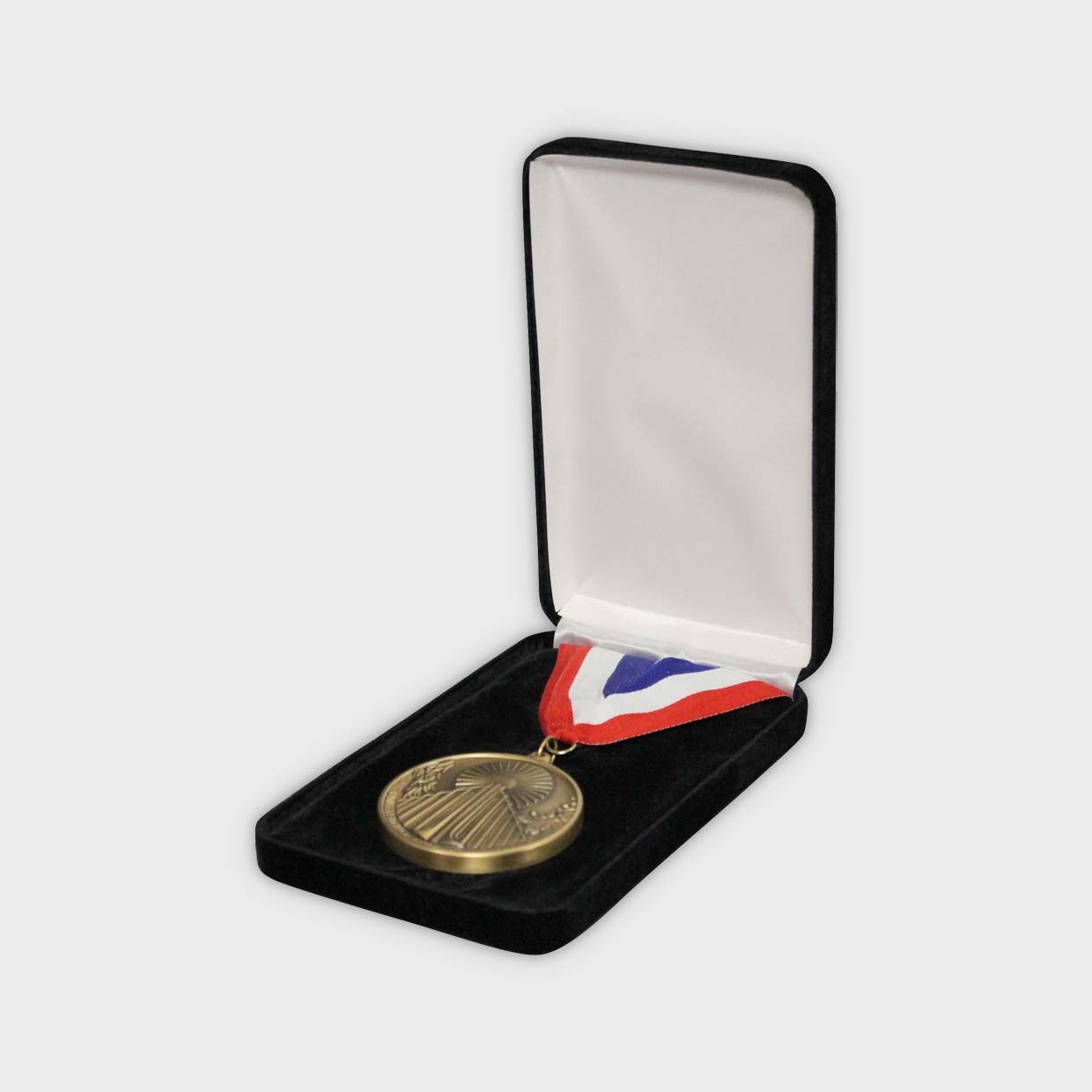This indoor photograph features a gold medal displayed in a black jewelry box, which is placed on a white table with a white background. The open box reveals a white cloth lining on the top and a velvet bottom. The medal, which prominently occupies the center of the image, is gold in color and is attached to a red, white, and blue ribbon. The medal itself appears to have a design that resembles a sun with a road extending from it, though no identifying information such as the event, year, or recipient is provided. The meticulous presentation and the professional setup suggest that the item might be intended for sale, auction, or exhibit.